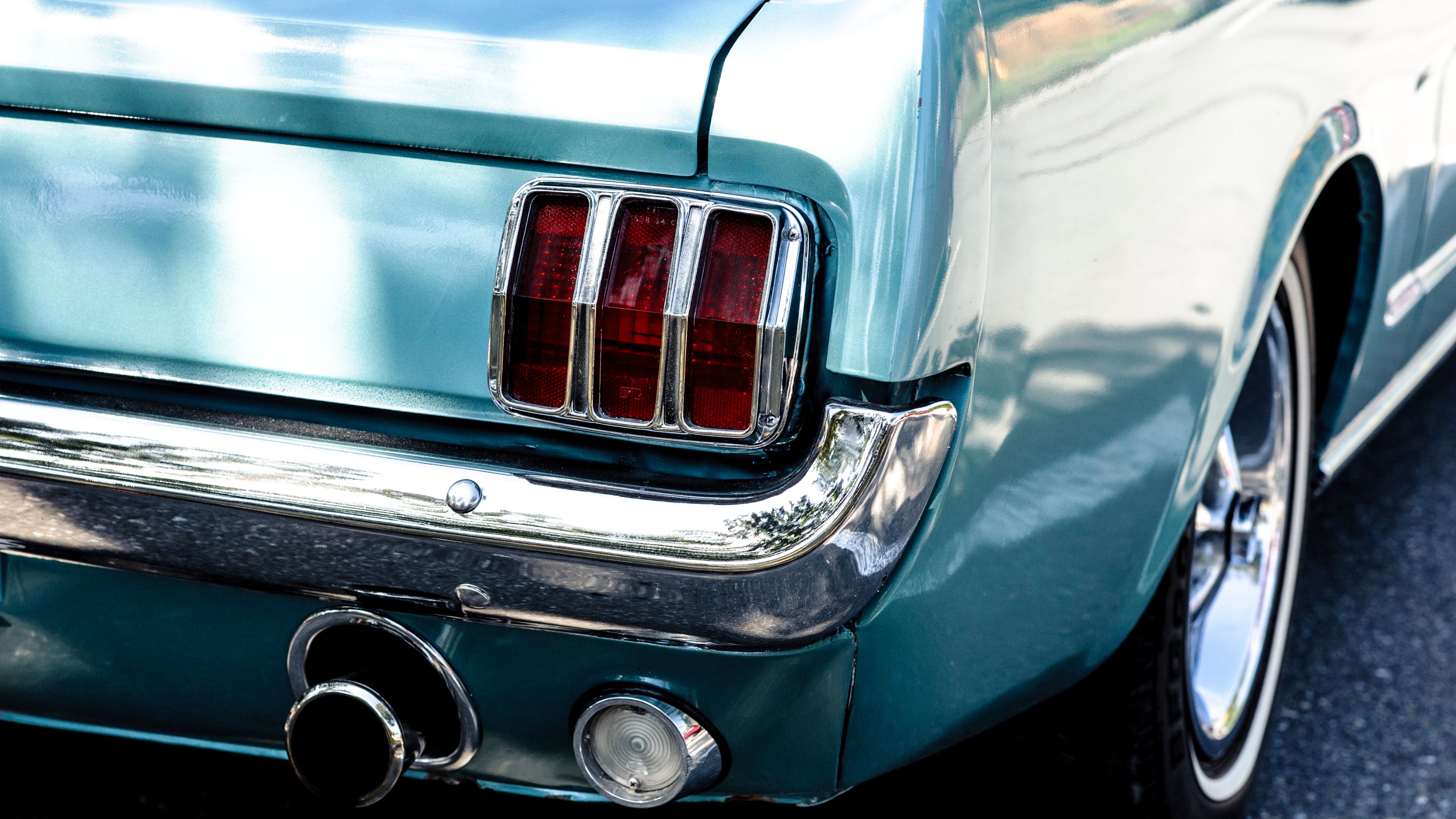The photograph captures a close-up of the rear end of a vintage, light blue car, likely a 1960s or early 70s Ford Mustang. Prominently featured are the car's distinctive three vertical, red taillights, each edged with chrome trimmings. The car's tailgate and bumper are also chrome, reflecting a shiny, polished finish. The lower edge of the image showcases chrome exhaust pipes situated in the center, with shadows—likely from a nearby tree—cast upon the vehicle. On the right side of the image, a black tire with a chrome rim is visible. The overall setting highlights the vehicle's classic automotive design, with attention to its gleaming silver elements and signature style.